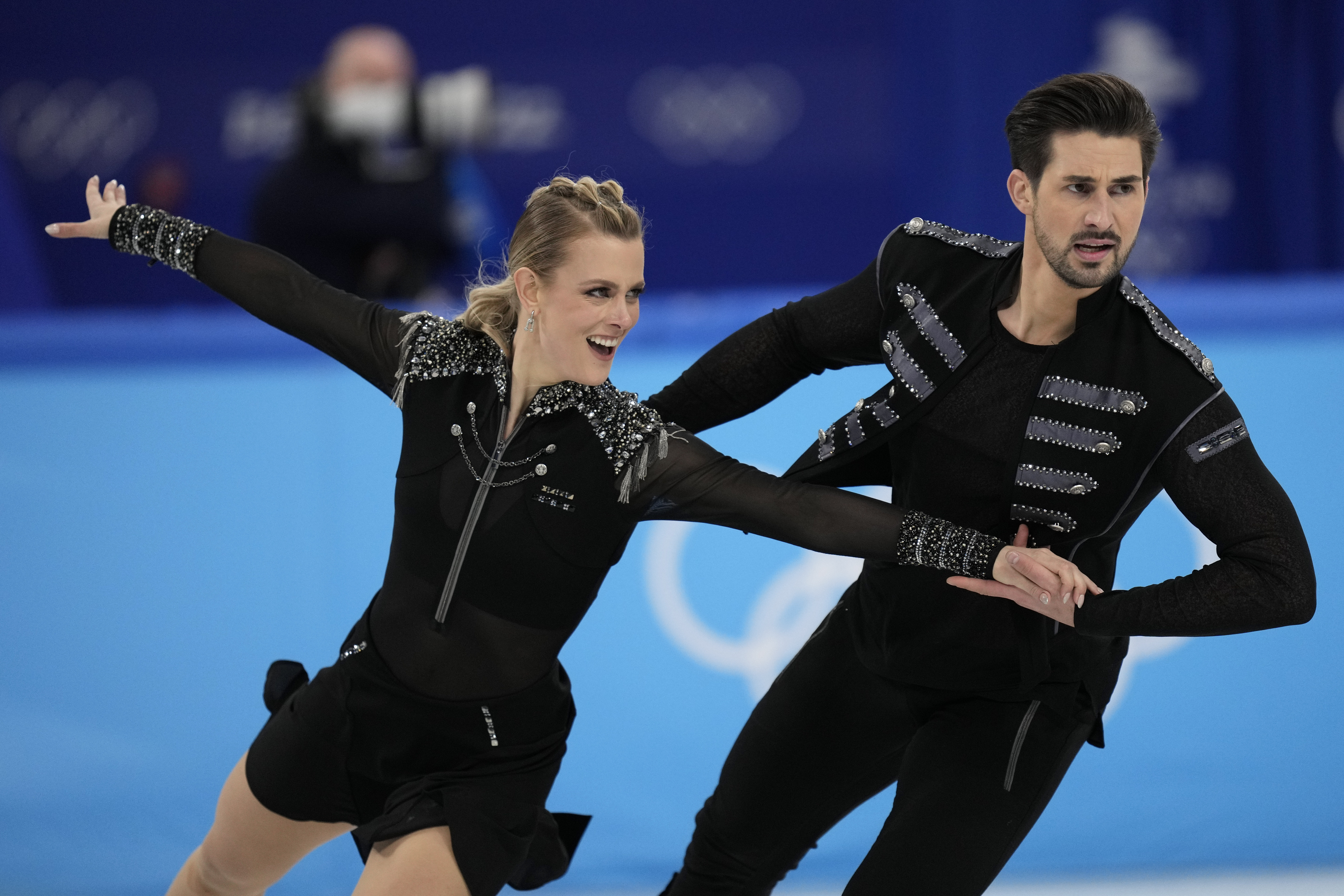The image depicts a couple performing in an ice skating competition, likely at the Winter Olympics, as suggested by the Olympic rings visible on a blurred dark blue and light blue background. The male skater is on the right, dressed in long black pants and a long-sleeved black shirt with a vest adorned with horizontal silver stripes and shoulder detailing. He has black hair and a subtle beard and mustache. The female skater is on the left, wearing a long-sleeved black top that transitions into a skirt decorated with silver tassels, sparkly jewels, and detailed cuffs. Her straight blonde hair is styled into small bows down the top center, pulled back into a ponytail. They are both Caucasian and are skating at an angle to the right, with the man holding the woman's left hand with his left hand. Her right arm is extended behind her, and she is smiling enthusiastically, while his right arm is also extended behind him. In the blurred background, a person wearing a mask, possibly their coach, can be seen observing the performance. The image is a rectangular photograph, capturing the skaters from the knees up as they glide gracefully on the rink.